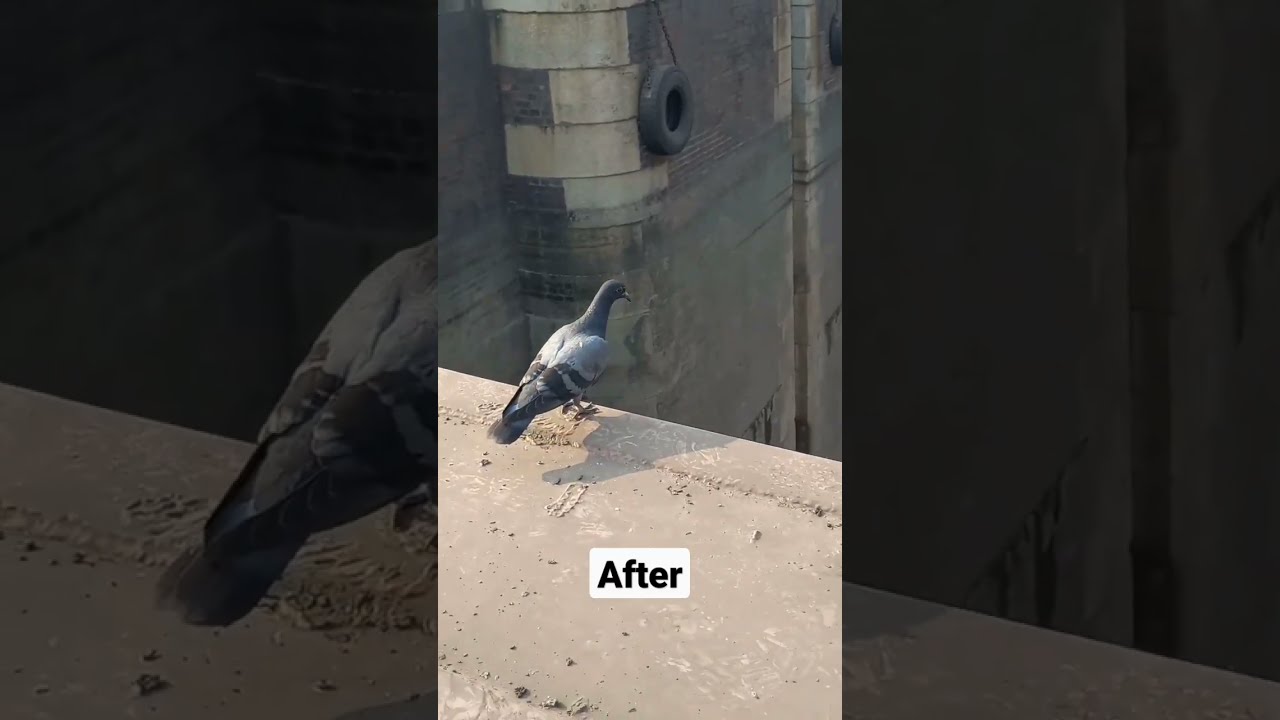In a portrait-oriented photograph seemingly taken with a cell phone, a single pigeon perched on the edge of a cement wall captures attention. The pigeon is positioned left of the image's center, its back to the viewer while it gazes downward towards the top right. The wall, composed of large beige and whitish stone pieces, features rounded pillars and has a rugged texture suggesting age and solidity. In the background, other elements of the structure come into view, resembling a castle or fortress with possible industrial traits. Notable are the black rubber tires tied to the wall, possibly serving as dock fenders. The pigeon itself has a distinct appearance with a gray head, white-marked wings, and a black tail with black stripes on the lower wings. The scene is set against an additional detail, a reflective water surface, further indicating the possibility of a waterfront area. At the bottom of the photograph, a white text box with black lettering reads “after.”